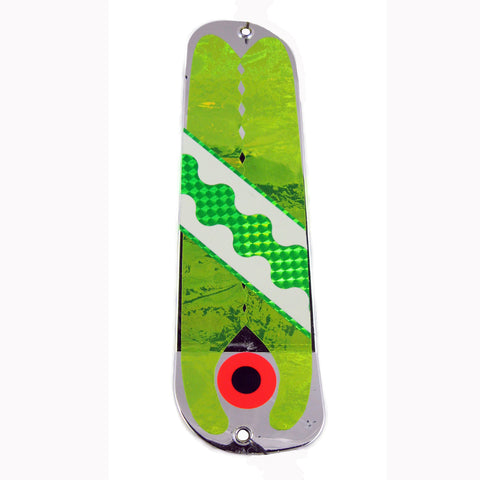The image shows a vertical skateboard-like object with a distinctive oblong, rectangular shape that curves at both ends. The board is predominantly green, featuring a textured green surface that extends across its entirety. The top and bottom edges of the board are silver and contain holes. Towards the base of the skateboard, there is a prominent bullseye design, with concentric circles—an outer red circle and an inner black circle. Diagonally across the center of the board, a white strip intersects the green texture, within which lies a detailed checkered pattern made up of light green and dark green squares. The sides of the board display hints of grey, creating a contrasting border around the green central area.